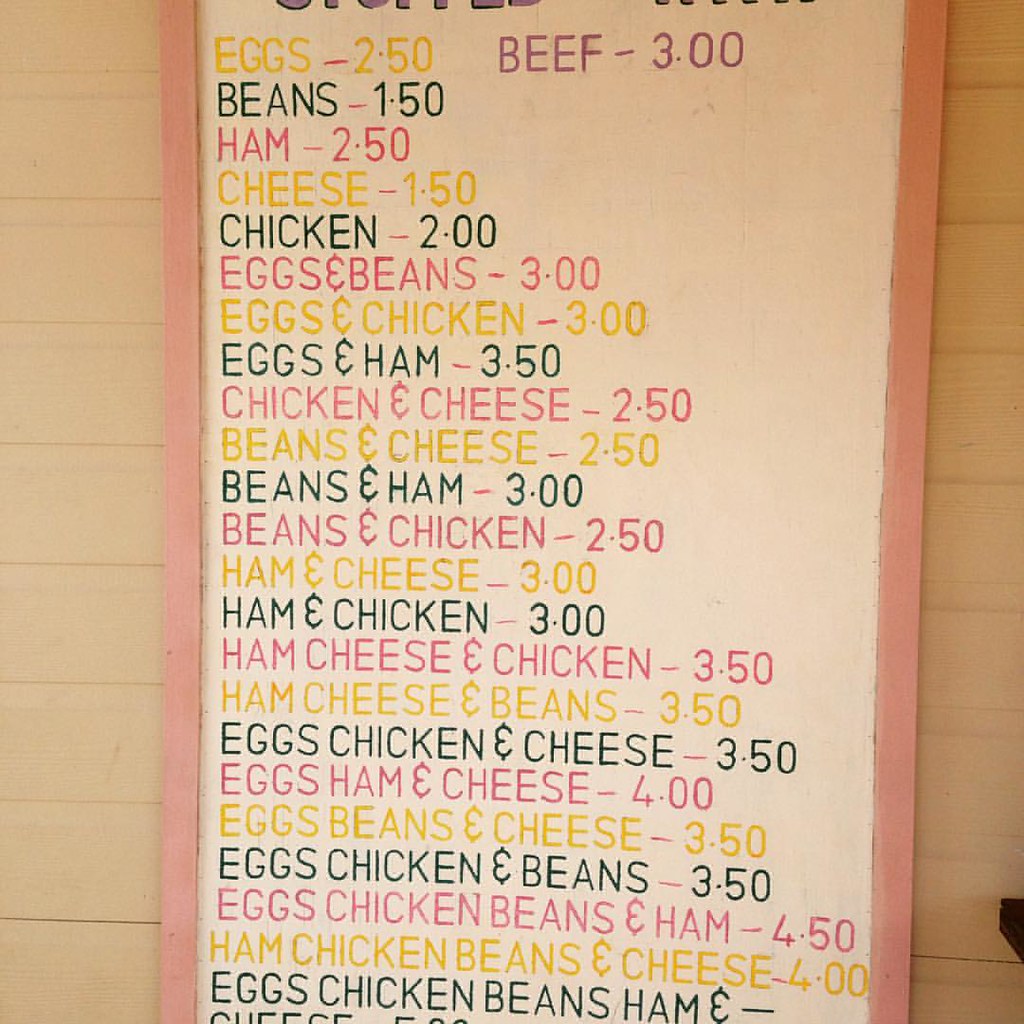The image features a long, vertical menu written on a rectangular sign with a white background and a dark pink border. The sign is mounted against a wall with very light yellow siding. While the very top portion of the menu is not visible, the remaining content is clearly written in a combination of yellow, pink, and black text. 

The menu items and their prices are as follows:

- Eggs: $2.50
- Beef: $3.00
- Beans: $1.50
- Ham: $2.50
- Cheese: $1.50
- Chicken: $2.00

Combination dishes include:
- Eggs and Beans: $3.00
- Eggs and Chicken: $3.00
- Eggs and Ham: $3.50
- Chicken and Cheese: $2.50
- Beans and Cheese: $2.50
- Beans and Ham: $3.00
- Beans and Chicken: $2.50
- Ham and Cheese: $3.00
- Ham and Chicken: $3.00
- Ham, Cheese, and Chicken: $3.50
- Ham, Cheese, and Beans: $3.50
- Eggs, Chicken, and Cheese: $3.50
- Eggs, Ham, and Cheese: $4.00
- Eggs, Beans, and Cheese: $3.50
- Eggs, Chicken, and Beans: $3.50
- Eggs, Chicken, Beans, and Ham: $4.50
- Ham, Chicken, Beans, and Cheese: $4.00

At the bottom, it appears to list "Eggs, Chicken, Beans, Ham, and Cheese" with a partially visible price, which looks like $5.00, though the text is somewhat cut off.